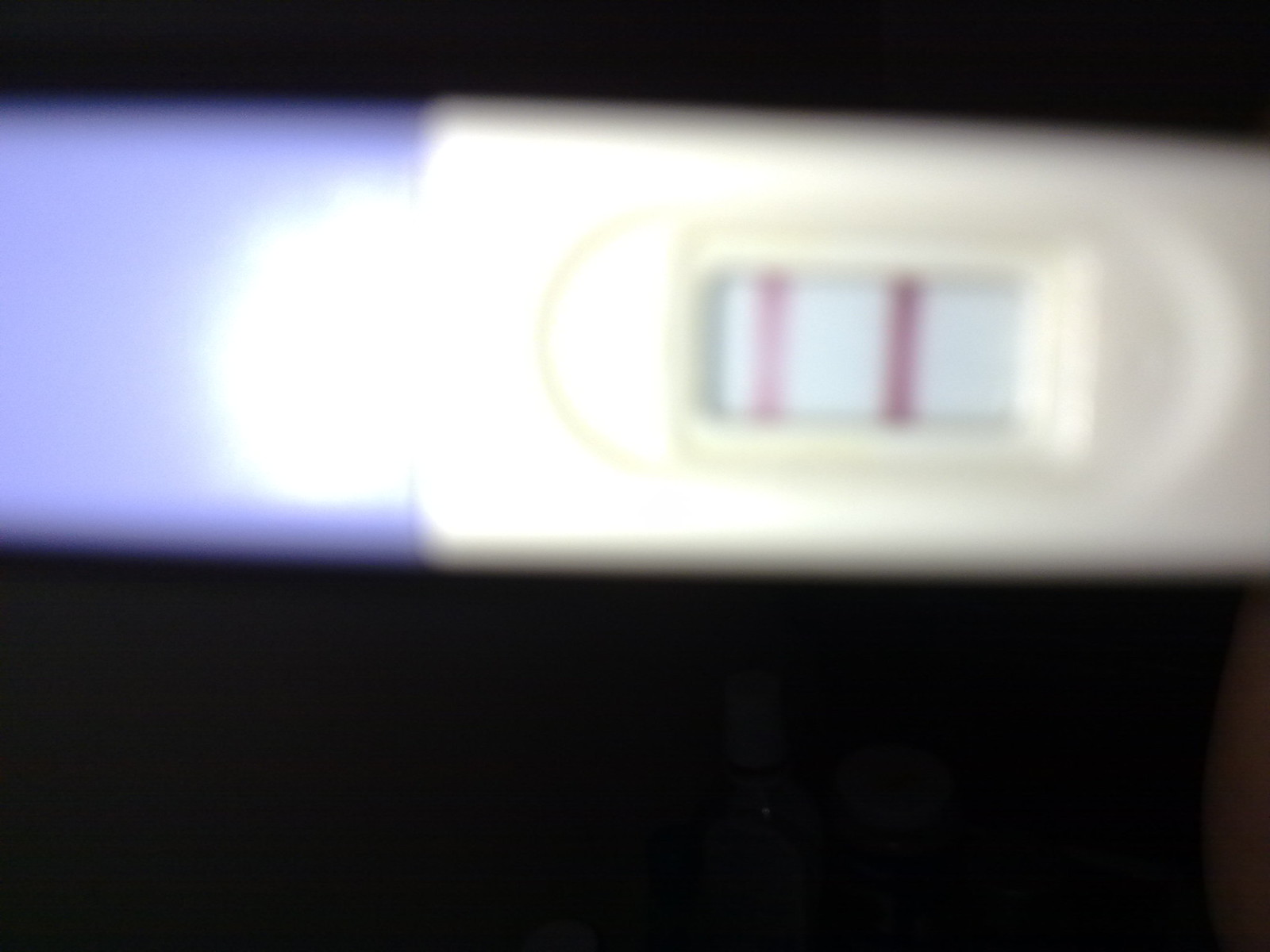The image features a pregnancy test held horizontally against a solid black background, likely taken with a flash. The test unit, which is beige in color, has a light blue-colored lower area on the left side. Despite the overall photo being out of focus, there's enough detail to note the test's readout window displaying what seems to be a positive result. The readout window, silver-gray in color, shows one darker vertical line towards its center and a lighter second indicator line towards its left, confirming the positive result. The key elements - the test unit, readout window, and background - are emphasized by the stark contrast provided by the flash.